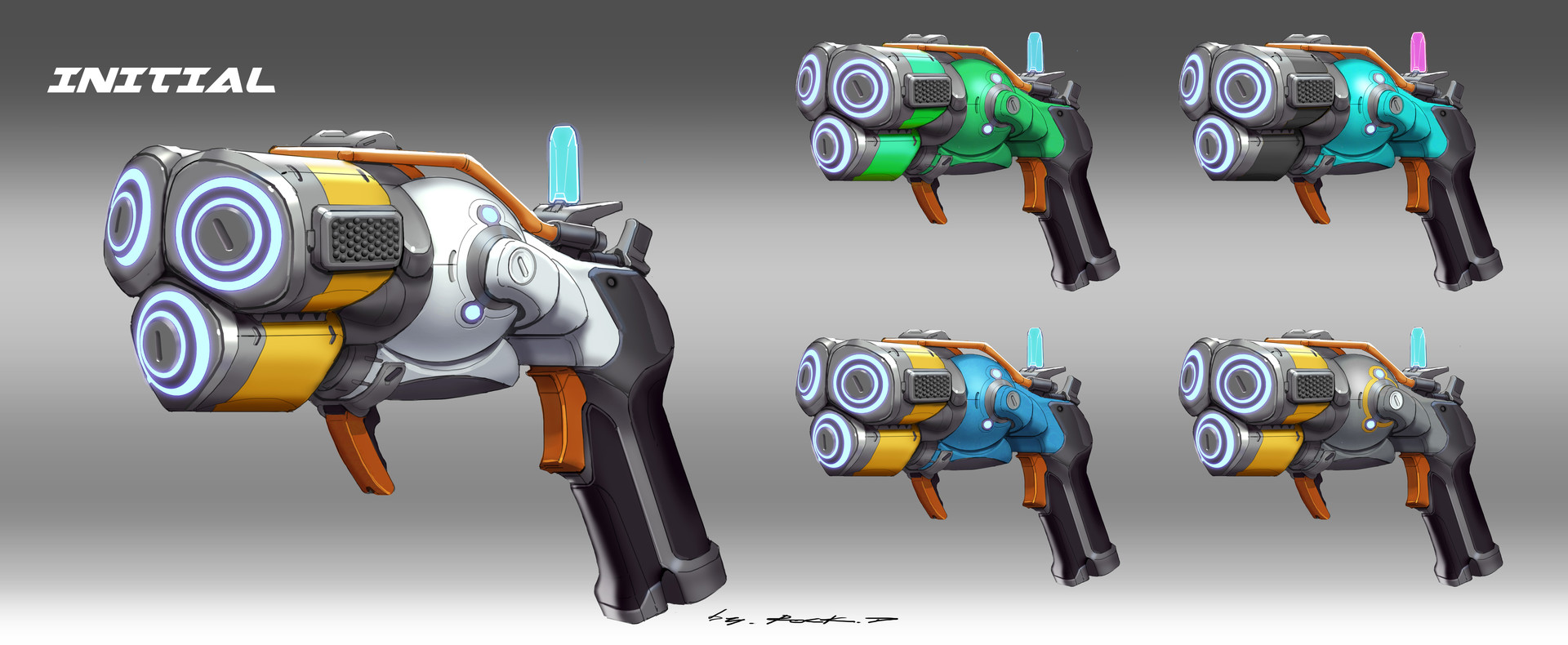This computer-generated image appears to be a rendering common on gaming websites, showcasing a fantasy-style handgun with distinctive and vibrant designs. In the upper left corner, the word "initial" is written in white letters against a grey background. The centerpiece is a large, detailed gun on the left, featuring three barrels arranged with two on top and one on the bottom. The barrels are primarily silver and yellow, with the gun's body adorned in white, black, and orange trim accents, and with a prominent black handle.

To the right, four smaller, computerized drawings depict variations of the same gun design, each with different color schemes. The first gun is green, black, and brown; the second is teal blue, brown, and black; the third is sky blue and yellow; and the fourth is dark gray and yellow. All these guns share the unique triple-barrel feature, with some descriptions noting that the barrel ends appear designed for key-like mechanisms, adding to the fantasy element. Finally, at the bottom middle of the image, there is a signature, attributing the artwork to its creator.